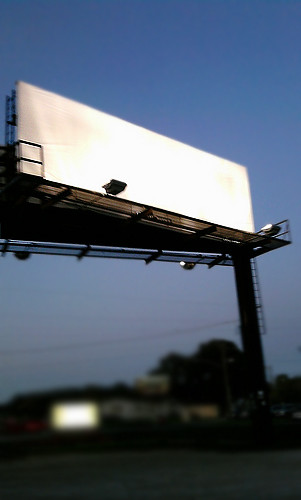The image features a blank, white billboard at street level, set against a backdrop of buildings and illuminated lights. The scene is anchored by a thick metal pole on the right side, equipped with a ladder that ascends to the billboard platform. At the platform, the structure forms a narrow V-shape, supporting billboards on each side. Visible scaffolding houses lights designed to illuminate the billboards. The sky above is cloudless, with the ambient light suggesting that the photo was taken near sunrise or sunset, adding a serene quality to the urban setting. Notably, the billboard lacks any advertising content or rental information, leaving it completely blank.